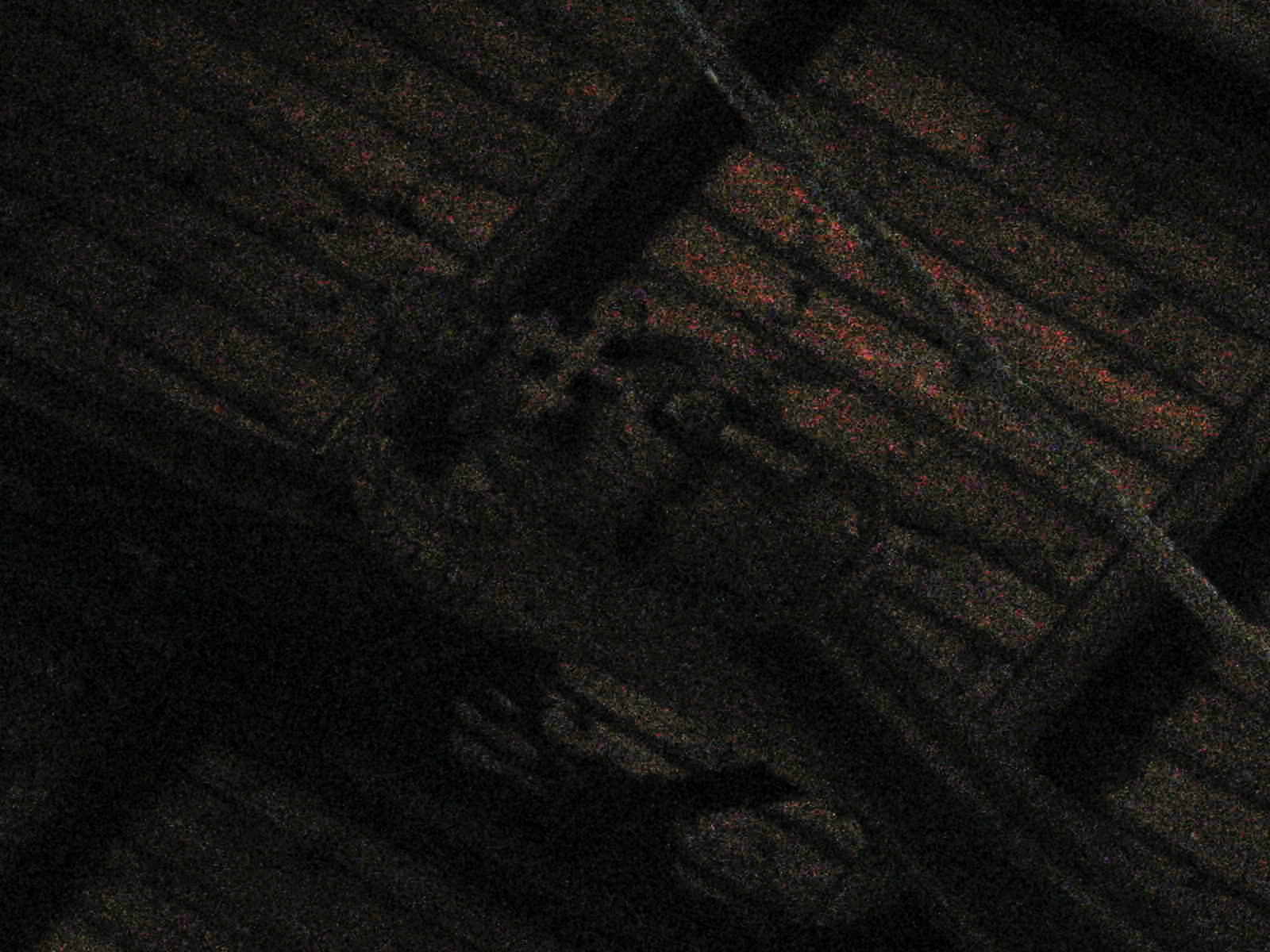In this grainy nighttime photograph, the primary colors are dark brown and black, enveloping an enigmatic scene. Dominating the frame, a statue emerges from the bottom right corner, extending diagonally towards the upper left. The statue appears to depict a woman draped in a flowing dress, her face faintly discernible in the low light. She is solemnly holding a cross with both hands in front of her body, exuding a sense of reverence or prayer. Adjacent to her figure, a stick or staff stands independently, leaning towards her side, adding to the mysterious atmosphere of the image. Despite the obscured details, the interplay of shadows and shapes invites a deeper contemplation of the scene.